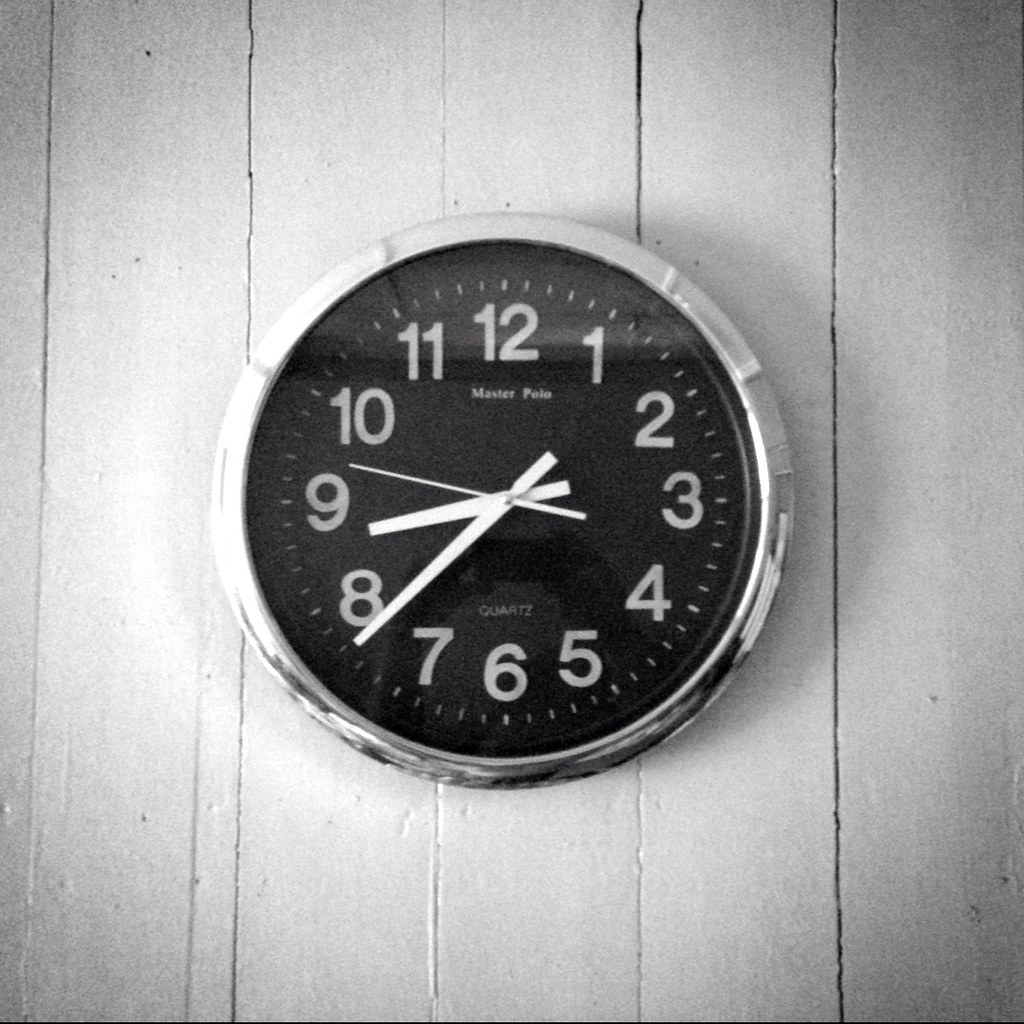The black-and-white image features a round clock mounted on a wall composed of wooden boards painted in a light color. The clock, framed with a shiny silver ring, has a black face with bold white Arabic numerals from 1 to 12 and minute hash marks around the edge. The clock showcases three white hands: the shorthand pointing between 9 and 8, the long hand between 8 and 7, and the second hand between 9 and 10. The face of the clock prominently displays the text "Master Polo" beneath the number 12, and "quartz" at the bottom. A glass cover protects the clock's surface and interior mechanisms.